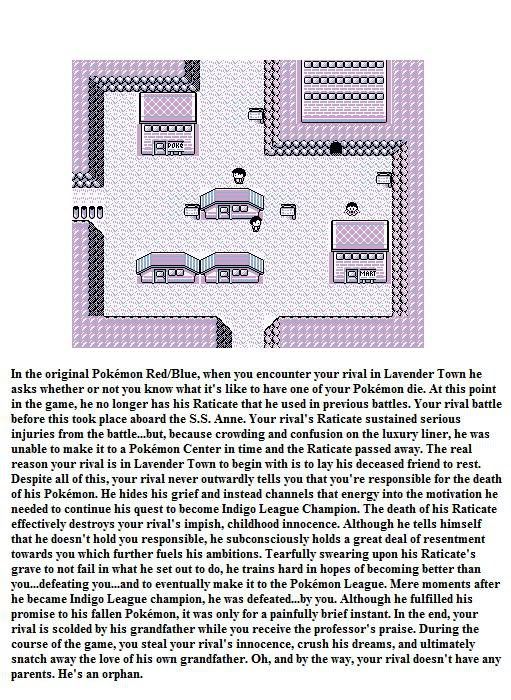This image depicts a moment from the original Pokémon Red and Blue games, set in Vermilion City. The backdrop features a distinct purple shade, adding a nostalgic hue to the scene. On the left side of the image, an L-shaped pathway can be observed, continuing towards the top and bottom edges of the frame. A prominent building is situated on the right side. In the top left corner, a Pokémon is visible, while another Pokémon can be seen in the bottom right corner.

Three flat, single-story buildings are also present, each characterized by one door and two windows. These buildings are strategically positioned: one in the middle, one at the bottom left, and one at the bottom middle of the image. Within this detailed setup, three human characters and three signs are scattered throughout the scene.

The context of the image ties back to a well-known Pokémon fan theory regarding your in-game rival's Raticate. The theory proposes that after a battle aboard the SS Anne, your rival's Raticate sustained injuries and, due to the chaos aboard the ship, could not reach a Pokémon Center in time, leading to its demise. The next encounter with your rival takes place in Pokémon Tower, a burial site for Pokémon, where he cryptically references the loss, fueling speculation and fan theories about his grief and motivations.

Beneath this visual tableau, extensive blocks of text provide additional narrative and theories, particularly focusing on the conspiracy that paints your in-game rival (often referred to as Gary) as a deeply affected character hiding his sorrow behind a façade of rivalry and aggression. The text delves into fan interpretations that suggest his actions are driven by an underlying grief over the loss of his beloved Raticate.

Note: The original text provided also contains colorful commentary and language which has been omitted for a more neutral, descriptive caption.